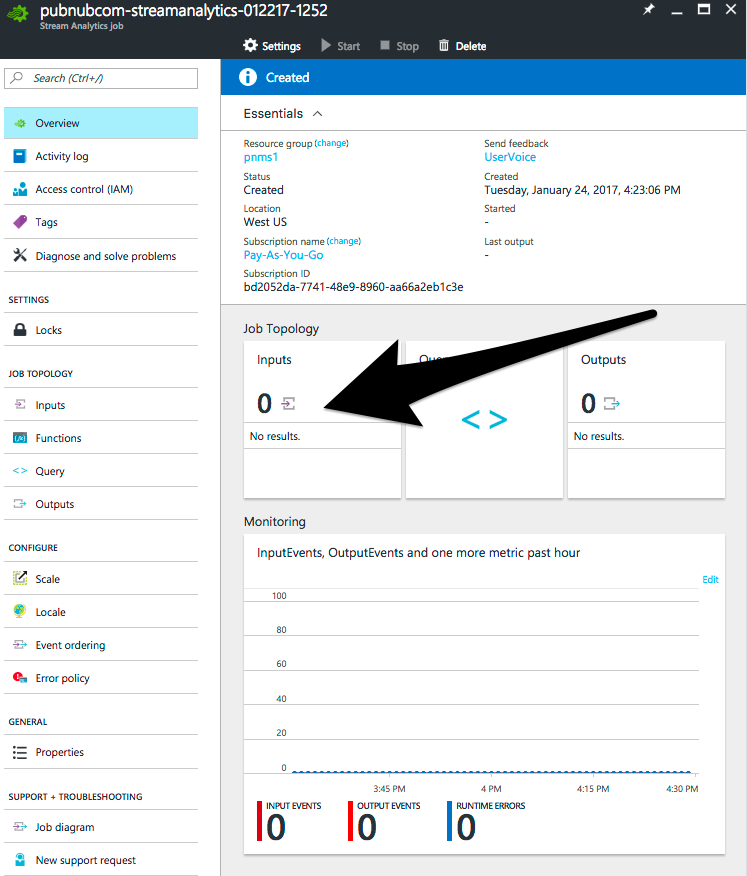**Detailed Description of the Screenshot:**

The screenshot showcases the Stream Analytics admin interface on the PubNub website (pubnub.com), specifically within the settings section. The interface features a large, text-oriented design with a prominent black horizontal menu bar at the top. The options on this top menu include "Settings" (where the user is currently located), "Start," "Stop," and "Delete."

On the left side, there is a comprehensive vertical menu offering various navigation options such as: 
- Overview
- Activity Log
- Access Control
- Tags
- Diagnosis
- General Settings
- Job Topology
- Inputs
- Functions
- Query Outputs
- Scale
- Locale
- A few other miscellaneous settings

To the right of the vertical menu, detailed system information and configuration options are presented. The essential information highlights that the resource group is named PMS1. Additional details include the feedback mechanism via User Voice, the creation date and time which is January 24, 2017, at 4:23 PM and 6 seconds, location in the Western US region, and that the subscription is on a Pay-as-You-Go basis. There is also a long alphanumeric subscription ID displayed for reference.

The Job Topology section is emphasized with a large black arrow overlaid on the image. This section currently indicates zero inputs and zero outputs, with no results.

Beneath this, a monitoring graph is presented, tracking metrics for inputs, outputs, and runtime errors. The timeline on the graph spans from around 2:45 to 4:30. The graph uses three distinct color codes: dark red, bright red, and blue. However, all metrics flatline at the bottom, indicating zero activity or errors during the given time frame.